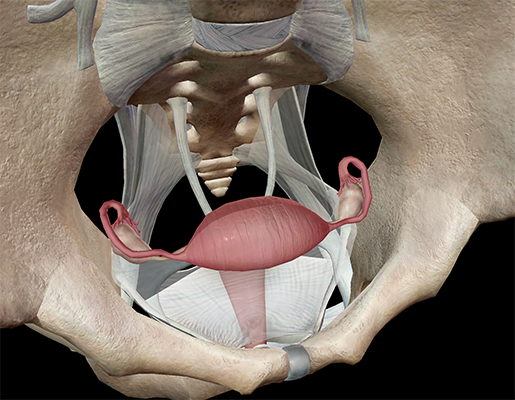The image depicts a detailed 3D rendering of the internal pelvic region of a female human, viewed from below. The skeletal structure, shown in cream or whitish hues, includes the hip bones, vertebrae, rib cage, shoulder blades, and spinal cord with visible sacrum and sacral parts of the tailbone. In the center, the pink reproductive organs—the uterus, ovaries, and fallopian tubes—are prominently displayed. These organs appear lifelike and soft compared to the more rigid, plaster-like appearance of the bones. Additionally, there are ligaments and tendons illustrated in a stark, whitish color, adding to the anatomical details of this cross-sectional view of a woman's pelvis.